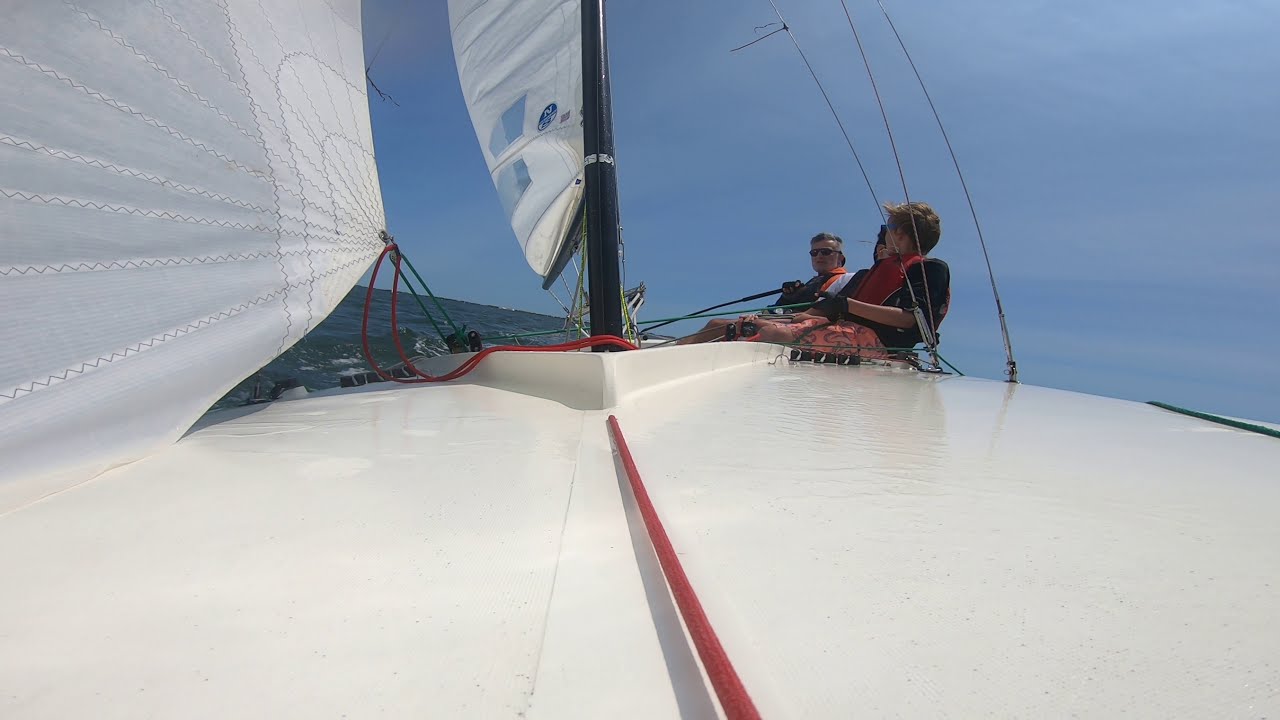This photograph, taken from inside a white sailboat, captures the vessel sailing in the open ocean with clear blue skies above. The boat features two white sails, one of which has indistinct blue writing. Several people, seen holding red ropes to navigate the boat, are on board, with two or three individuals visibly seated. They are wearing life vests for safety as they direct the sailboat through the dark blue, relatively calm ocean waters, with only small waves breaking the surface. The atmosphere appears tranquil, with the sky a deep blue and nearly cloudless, suggesting a beautiful day for sailing.